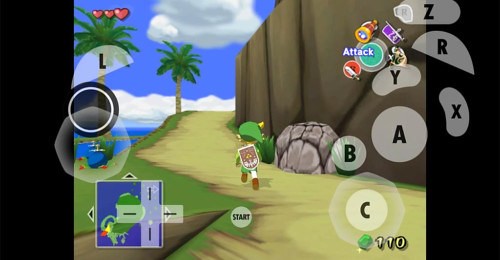A vibrant screenshot from a video game captures an adventurous coastal beach scene, presented in landscape widescreen orientation with thick black margins framing the sides. The character, adorned with a green hat and a shield on their back, strolls along a sandy path that winds beside a serene blue sea. Under a clear blue sky, two palm trees sway gently, adding to the tropical ambiance. The top of the screen displays various infographics, with a small map showcased in the bottom left corner and some black letters surrounded by a white, slightly opaque background on the right. Other small infographics representing in-game items are scattered across the interface. In the top left corner, three hearts indicate the character's health status.